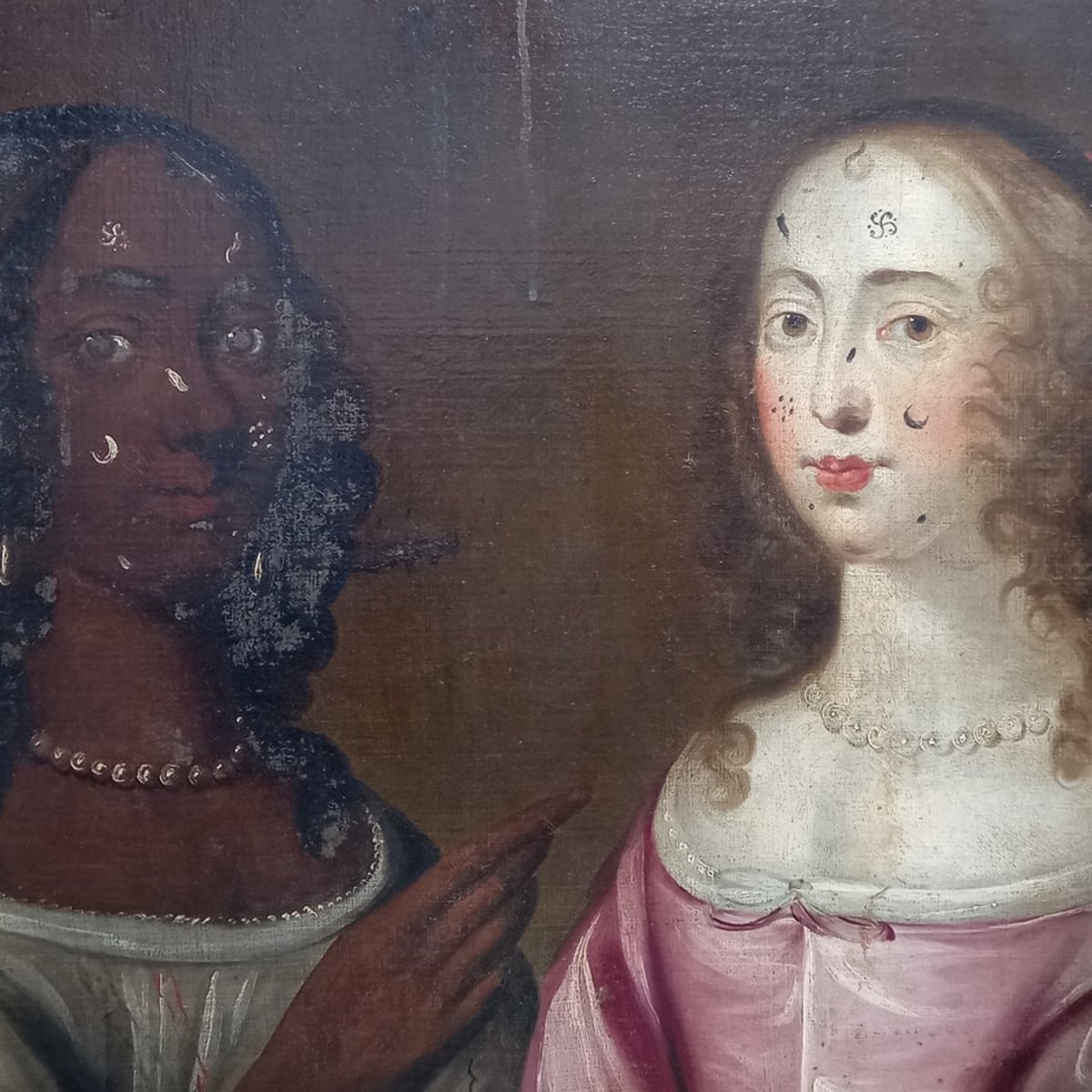The image showcases a detailed, square-shaped photograph of a Victorian-style oil painting featuring two distinct women, partially cropped and zoomed in. Both women are visible from the chest upwards, set against a dark brown background with noticeable paint drips. On the left is an African woman with dark skin, adorned in a green low-neckline dress and a black pearl necklace. She has long, black curly hair and is marked with white facial symbols, including a crescent and dots. To her right is a European woman with light skin, wearing a pink low-cut Victorian dress, complemented by a white pearl necklace. She similarly has facial symbols like a crescent moon and dots. Both women share matching shoulder-length hairstyles parted in the middle, smiling gently towards the viewer. The woman on the left has her right hand slightly raised, pointing towards her companion, adding a dynamic interaction in the composition.